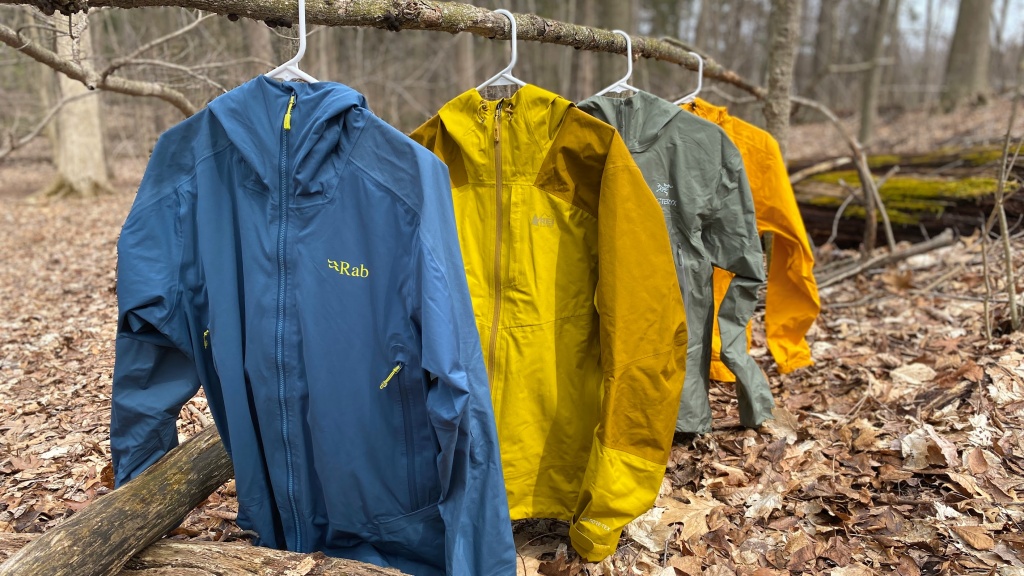In the heart of a dense, wintry forest, an artistic scene unfolds, reminiscent of a carefully staged advertisement. A robust, dead branch, fashioned into an impromptu closet pole, stretches horizontally amidst the leaf-strewn forest floor. Hanging from this branch are four lightweight, rainproof jackets, each displayed on white hangers. The jackets, seemingly from the same brand, are arranged in a row, closest to farthest from the camera, in striking colors: the first is a light blue jacket with "R.A.B." inscribed in yellow on the breast area and features a yellow zipper, the second is a vivid yellow jacket, the third a light gray jacket, and the last a vibrant orange jacket with a slightly more intense hue than the second. The jackets contrast sharply against the natural backdrop of leaf-covered ground interspersed with fallen logs, some draped in green moss. Surrounding them are countless gray, leafless trees, creating a stark, photorealistic scene. The jackets, with their bright unnatural colors, look oddly out of place in this serene forest setting, capturing immediate attention amidst the tranquil, naturalistic lighting.